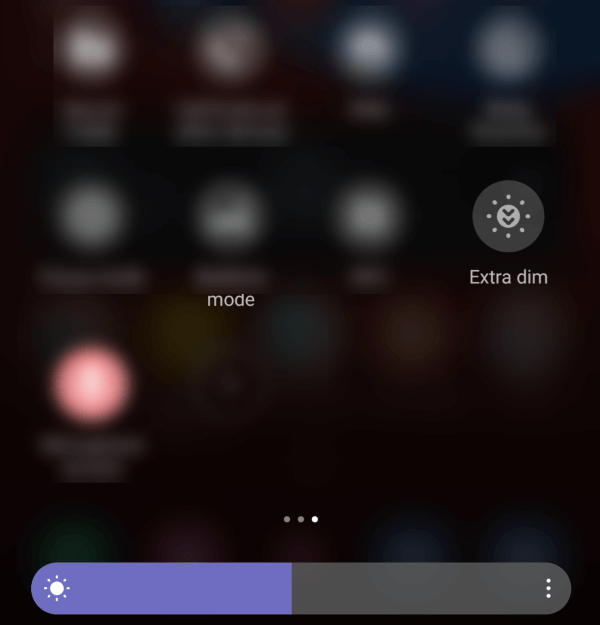This image showcases a screenshot of the brightness settings page on a cell phone, displayed as a vertical rectangle with a black background. The top row contains several app icons that are clickable; however, they are blurred out, appearing as slightly gray and out-of-focus images. Moving down, there is another row of four icons. The first three of these icons are also blurred out, but under the second icon from the left, the word "Mode" is visible in white text. The fourth icon on the right is more discernible, featuring a gray circle with smaller circles of dots within it. Inside this, there is a lighter gray circle with two downward-pointing arrows, and beneath this icon is the label "Extra Dim."

Continuing downwards and to the left, there is another blurred app icon that appears to have pink and white colors. At the bottom of the page, there is an oblong brightness adjustment bar. On the left side of this bar, there is a blue icon of a sun, and to the right of this icon, there are three vertical white dots. The right side of the brightness bar is dark gray, completing the user interface for adjusting screen brightness settings.